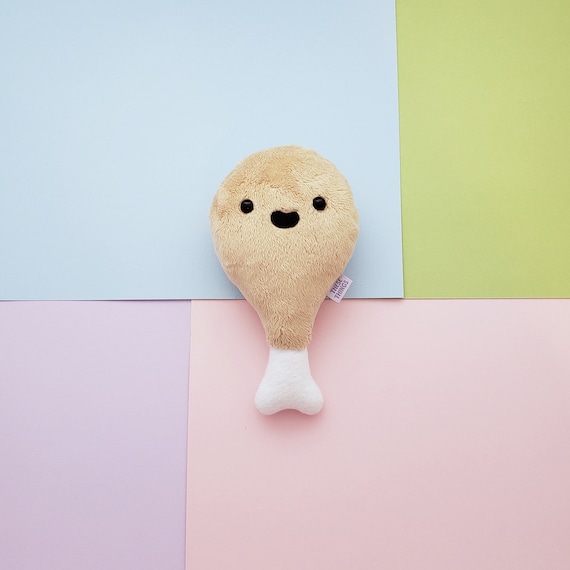The image shows an up-close view of a squishy, plush toy shaped like a chicken drumstick. The plushie is crafted from light brown velvety fabric, emulating the drumstick's meat, and a white fabric for the bone, which gives it the appearance of standing upright on its end. The toy features a cute, cartoon-like face with two black bead eyes and a small black smile. It is set against a colorful background comprising four pieces of construction paper: cyan blue in the top left, forest green in the top right, pink in the bottom right, and purple in the bottom left. A small tag is attached to the plushie, possibly containing washing and care instructions. The drumstick toy is the central focus of the image, highlighted by the contrasting vibrant construction paper layers.